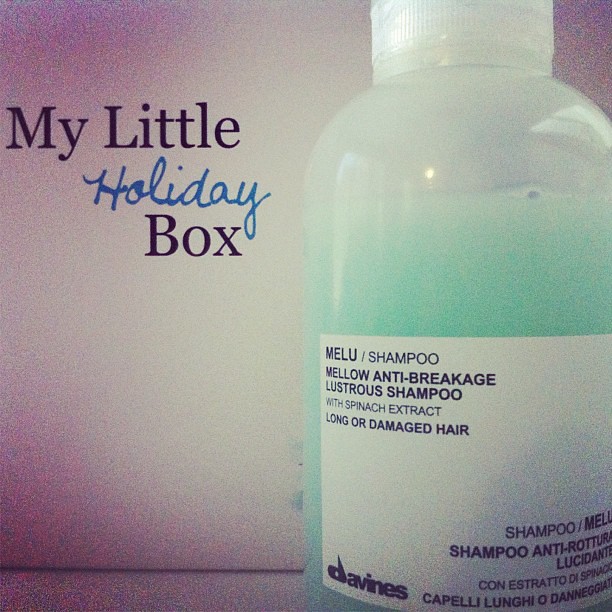The image is an advertisement for Melu shampoo set against a light tan backdrop with purple tints in each corner. On the left, there is a message reading "MY LITTLE HOLIDAY BOX," with "MY LITTLE" and "BOX" in black, capitalized letters, while "HOLIDAY" is handwritten in blue. Taking up the right side of the image is a semi-transparent plastic bottle containing a lavender-aqua green liquid and topped with a white cap. The bottle's label features the text "Melu shampoo" and describes it as a "mellow anti-breakage lustrous shampoo with spinach extract, for long or damaged hair." Beneath this, the brand name "Davines" appears on a white label, denoted with a trademark symbol. The label also includes additional information in what appears to be Italian: "concentrato capelli lunghi."